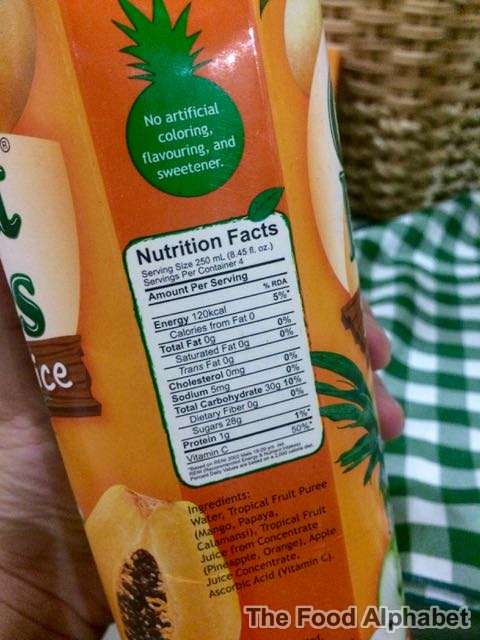In this image, we see a close-up of the side of a juice carton, specifically focusing on the nutrition label. The juice carton itself is a vibrant orange color, indicating it might be tropical or orange juice. Behind the juice carton, a green and white checkered blanket and a wicker picnic basket are visible, suggesting the scene might be set outdoors as a picnic. A person's hand is holding the orange juice carton, making the scene appear casual and spontaneous.

The nutrition label provides detailed information about the contents of the juice. It lists the ingredients as water, tropical fruit puree, tropical fruit juice, and sorbic acid. Additionally, the bottom corner of the label features the food alphabet, providing further nutritional context. The overall setting combines elements of a relaxed picnic atmosphere with an informative focus on the juice's nutritional content.